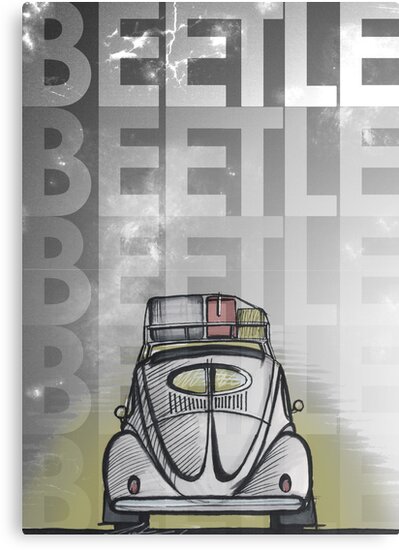This is a detailed and professional illustration of the back of a white Volkswagen Beetle car, rendered in a comic or cartoon style using pencil and ink. The car is prominently positioned at the bottom center of the image, turned away from us, showcasing its distinctive, round shape. On the roof of the car, there is a luggage rack holding three items—one white, one pink, and one yellowish. The background features a textured black-and-white sky. Overlaid across the sky are the words "Beetle," which appear in large letters at the top and gradually fade as they repeat five times down towards the bottom of the image. The only colors present in this artwork are black, white, yellow, red, and various shades of gray, highlighting its classic, old-school aesthetic.